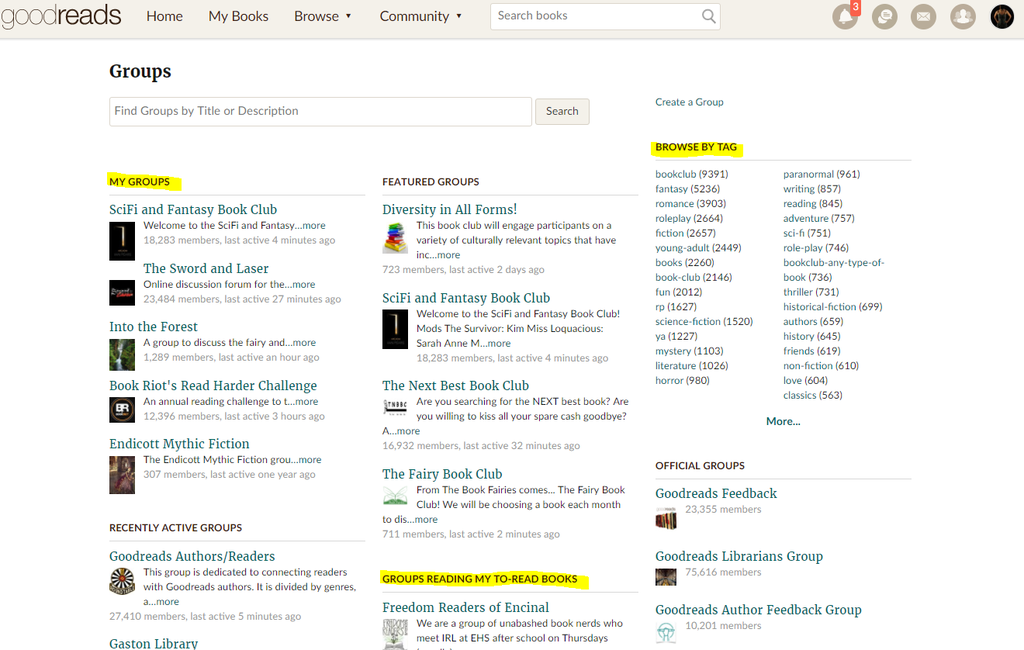This image is a screenshot from the Goodreads website. The overall background of the website is primarily white, providing a clean and minimalist appearance. At the very top, the website features a light tan-colored toolbar that spans the width of the page. In the top-left corner, the Goodreads logo is prominently displayed, consisting of the word "Goodreads" in a stylized font.

Positioned to the right of the logo are several navigational buttons, including "Home," "My Books," a dropdown menu labeled "Browse," and another dropdown menu labeled "Community." Further to the right is a white, rectangular search box, which has the placeholder text "Search books" on the left side and a small magnifying glass icon on the right.

Continuing along the top toolbar, there is a bell icon with a small red rectangle containing the number three, indicating three new notifications. Next to the bell icon, there are icons for messages (mail) and possibly an account or profile.

The main body of the webpage is dedicated to "Groups." Directly beneath the main header is another search box labeled "Find groups by title or description" with an accompanying search button. Below this search functionality, several groups are listed, categorized under headers such as "My Groups," "Groups Reading," "My To Read Books," and "Browse by Tag." These sections are highlighted with a yellow highlighter, drawing attention to key areas of interest.

The image captures the structured and user-friendly design of the Goodreads website, emphasizing its navigational features and group search functionality.